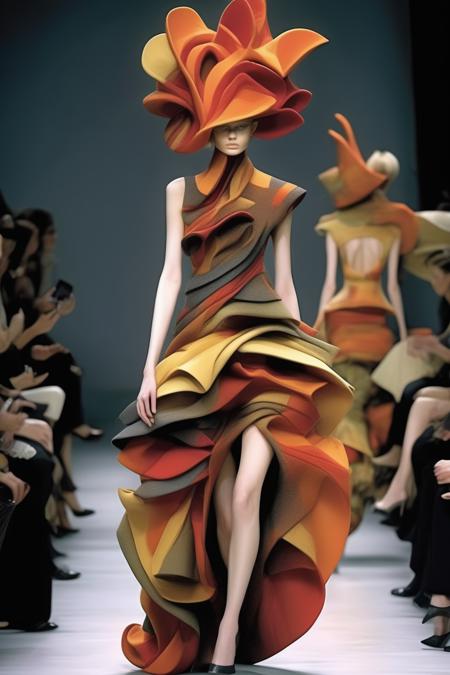The image captures an ethereal runway show, with models striding down a pristine white runway against a muted gray backdrop. The audience, seated in rows on either side, is partially visible, displaying glimpses of knees, legs, and the occasional curious face peeking forward. Many spectators are engrossed in capturing moments on their cell phones. The central focus is a striking female model advancing toward the camera. Her elongated, slender limbs are accentuated by her ivory, pale skin. She dons a dress adorned with an abundance of heavy ruffles, revealing much of her thighs and legs. The back of the dress transforms into a floor-length skirt composed of multiple layers of fabric in muted earth tones, such as burnt orange, yellow, brown, dark green, and rust-colored red. Her ensemble is crowned by an elaborate hat, featuring layers of fabric in oranges, yellows, and reds, resembling flickering flames. This vibrant headpiece adds a dramatic flair to her already captivating appearance.